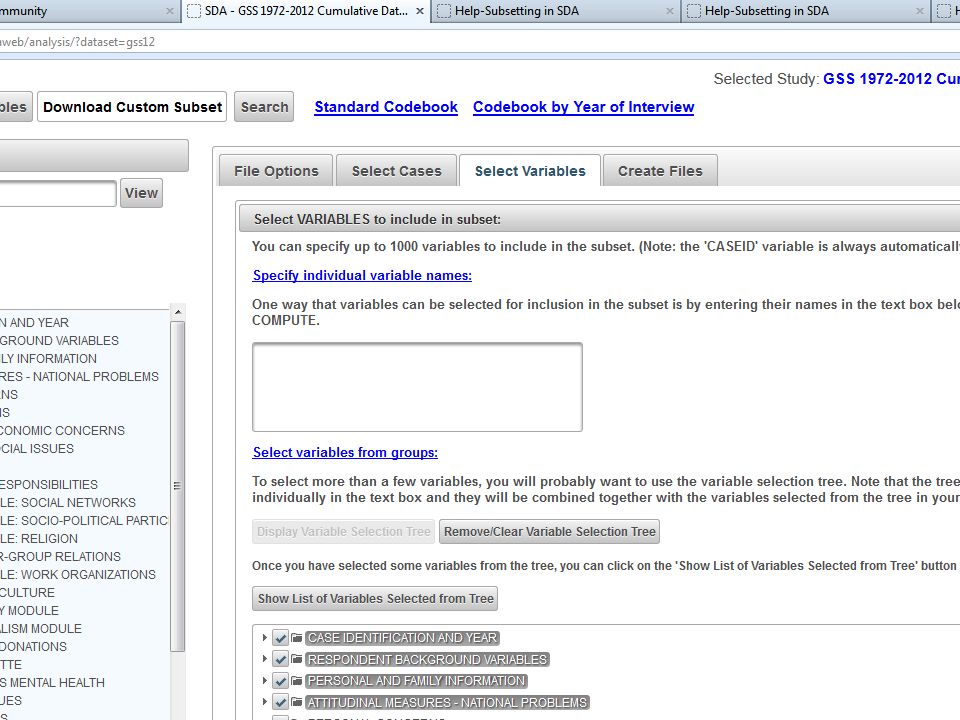The image is a detailed screenshot of a web interface displaying a selection area of a website. Positioned towards the middle of the screen are several sections labeled "File Options," "Select Cases," "Select Variables," and "Create Files." Specifically, the screenshot highlights the "Select Variables" section. 

In this section, instructions indicate that users can select variables to include in a subset, with a maximum of 1,000 variables allowed. Below this instruction is a prompt stating, "Specify variable names." This section explains that one way to select variables is by entering their names into a large text box provided below. Additionally, there is an option labeled "Select variables from group," followed by various selectable options.

The interface appears user-friendly, with a clean layout that guides users through the steps of selecting and specifying variables for their desired subsets.